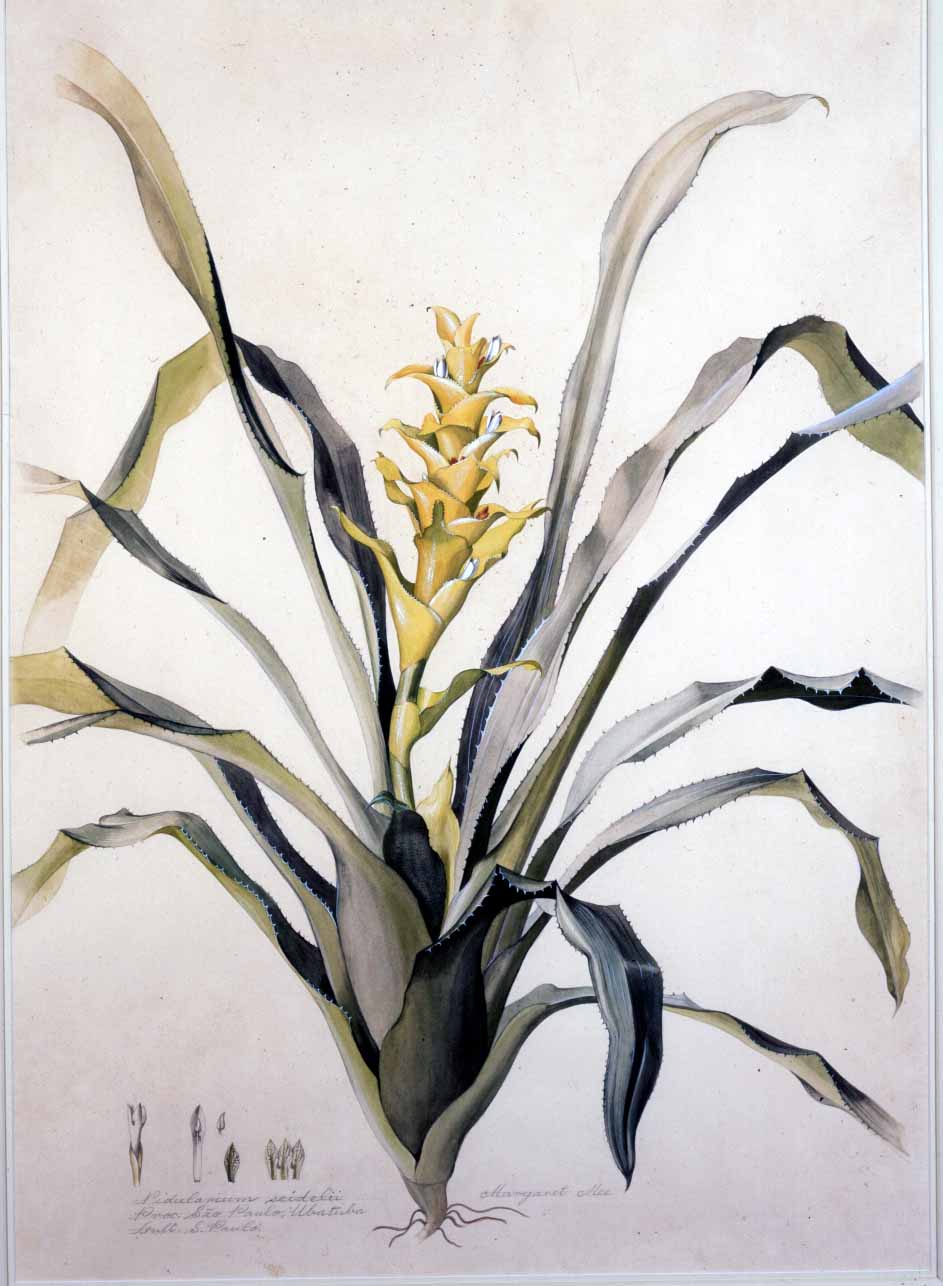This detailed illustration appears to be a watercolor painting, potentially from a book, depicting a flowering plant against an off-white background. The plant is shown with its roots embedded in the ground, extending upwards with large, green, gray, teal, and hints of light blue leaves. These leaves gradually arch over as they grow longer. At the center of the plant stands a prominent yellow bulb, resembling a plume, accompanied by levels of yellow petals sprouting along the stem. The artwork combines aspects of pencil illustration with watercolor, yet maintains a clean, solid appearance without typical watercolor bleeding. Below the plant, to the left, are smaller, less distinctive drawings of other plants, accompanied by three lines of minimal, difficult-to-read text. Additional text is found next to the illustration which may include the plant's name, but it is not legible. The predominantly muted color palette features shades of white, yellow, black, gray, light blue, and light green.